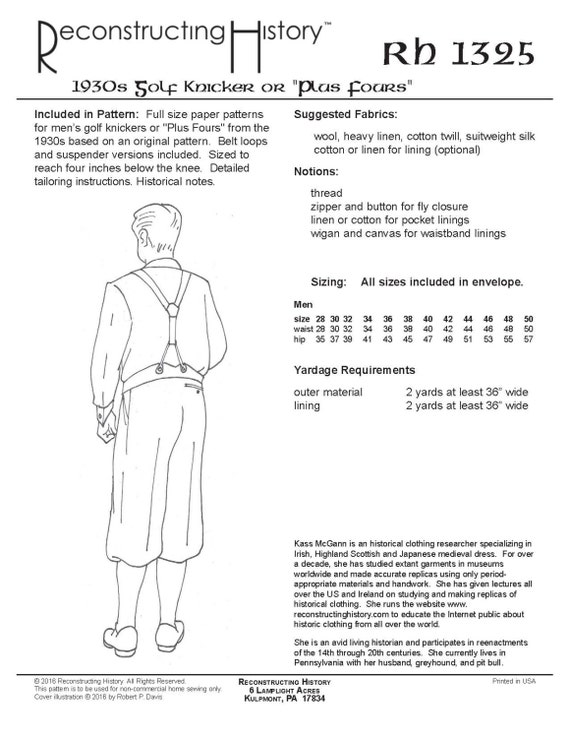The image shows a black and white poster or product label for a set of sewing patterns titled "Reconstructing History: 1930s Golf Knicker or Plus Fours (RH1325)." The poster features a detailed description of the patterns, which are full-size and based on original 1930s designs. These knickers are described as reaching four inches below the knee, available in both belt loops and suspender versions, and come with detailed tailoring instructions and historical notes. 

The patterns suggest using fabrics such as wool, heavy linen, cotton twill, suit weight silk, and cotton or linen for linings. It includes information on required notions, sizing, and yardage requirements. There’s a visible illustration of a man wearing the golf knickers with suspenders, showing a detailed view from the back. The suspenders meet at a central brace and split over the shoulders, and the knickers are gathered below the knee. 

At the bottom, there's contact information for "Reconstructing History" including an address at Lamp Light Acres, Kills Point, Pennsylvania, and a copyright notice from 2018, noting the product is printed in the USA. This appears to be an advertisement or guide for seamstresses interested in historical clothing patterns.